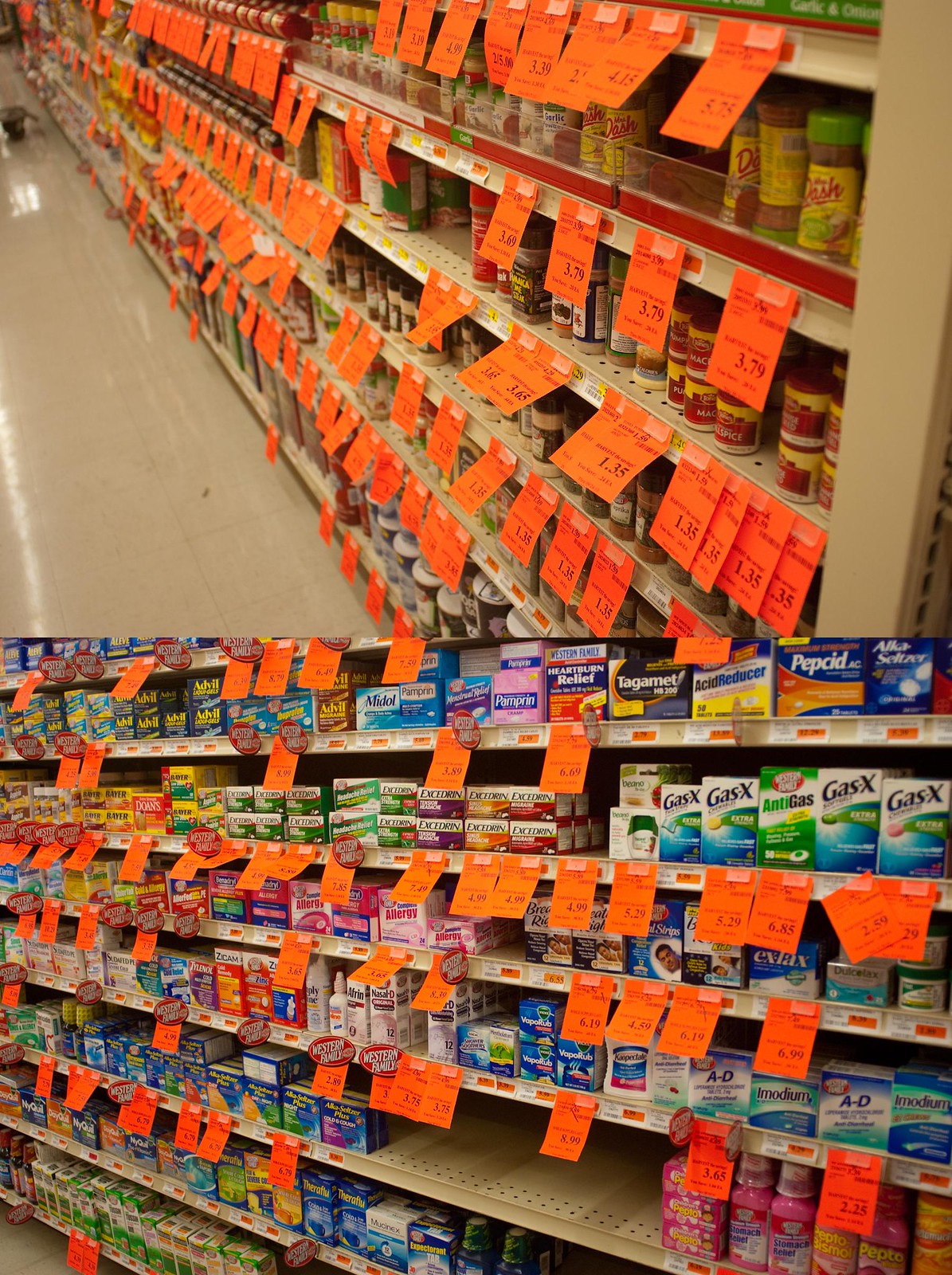The image captures a bustling aisle in a drugstore, neatly divided into two sections stacked vertically—a spice section above and a healthcare section below. The spice shelves are narrow, packed tightly with an array of seasonings, reflecting the typical setup in a grocery store. Below, the healthcare shelves, stocked with essentials like Gas-X, Tylenol, and Advil, extend across white, standard store shelving. The floor, which glimpses briefly in the spice section, boasts a shiny linoleum surface, enhancing the store's clean and sterile aesthetic. What immediately catches the eye are numerous bright orange sale tags dotting the shelves, resembling sticky notes hastily placed to announce special bargains. These striking tags contrast sharply against the white shelves, boldly presenting the savings available to shoppers and adding an energetic touch to the scene.